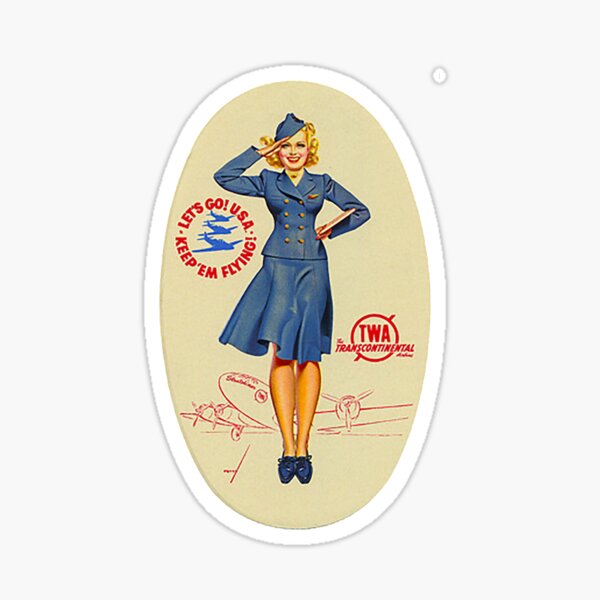This image depicts a vintage-style patch that is likely a badge or sticker associated with TWA (Transcontinental Airways). The oval-shaped patch has a beige background with a white border, featuring a nostalgic 1950s-1970s pinup aesthetic. In the center stands a young, white, blonde-haired woman dressed in a classic stewardess outfit: a blue uniform with a buttoned jacket, knee-length skirt, and matching shoes. She strikes a salute pose, with one arm raised to her forehead and the other resting on her waist.

To the left of the stewardess, the patch displays the slogan "Let's go USA, keep them flying," encircling three silhouetted airplanes. To her lower right, near her knees, it reads "TWA, Transcontinental." Behind her, a sketch of a TWA four-engine airplane is illustrated in red, though there appears to be an artistic inconsistency with the number of engines, giving it an AI-generated feel. The overall design of the patch exudes a retro aviation theme, complete with a stylized aircraft reminiscent of the mid-20th century.